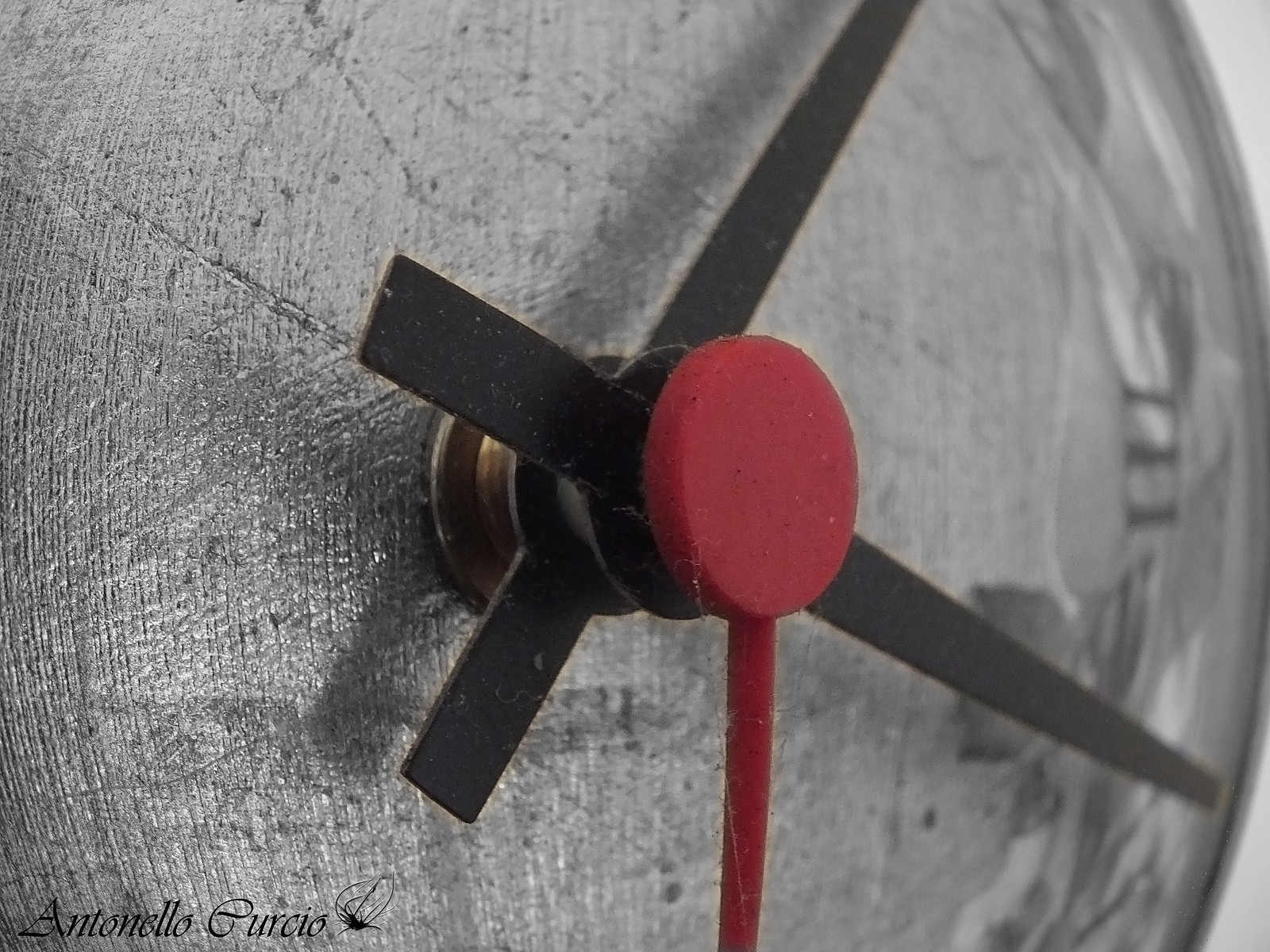In a crisply detailed, horizontally rectangular frame, the close-up image of a sophisticated silver clock face, captured at a slight angle from the 9 o'clock position, dominates the scene. The only visible numeral, a Roman numeral III, subtly stands on the right, adding a touch of classical elegance. The right side of the frame gently blurs, emphasizing the sharp clarity of the clock’s intricate center. The focal point is the point where the clock hands converge – the sleek black minute and hour hands, and the striking red second hand, which extends downwards, embodying precise craftsmanship. The signature "Antonello Curcio" subtly adorns the bottom left corner in black, adding an artist's mark to this refined composition.